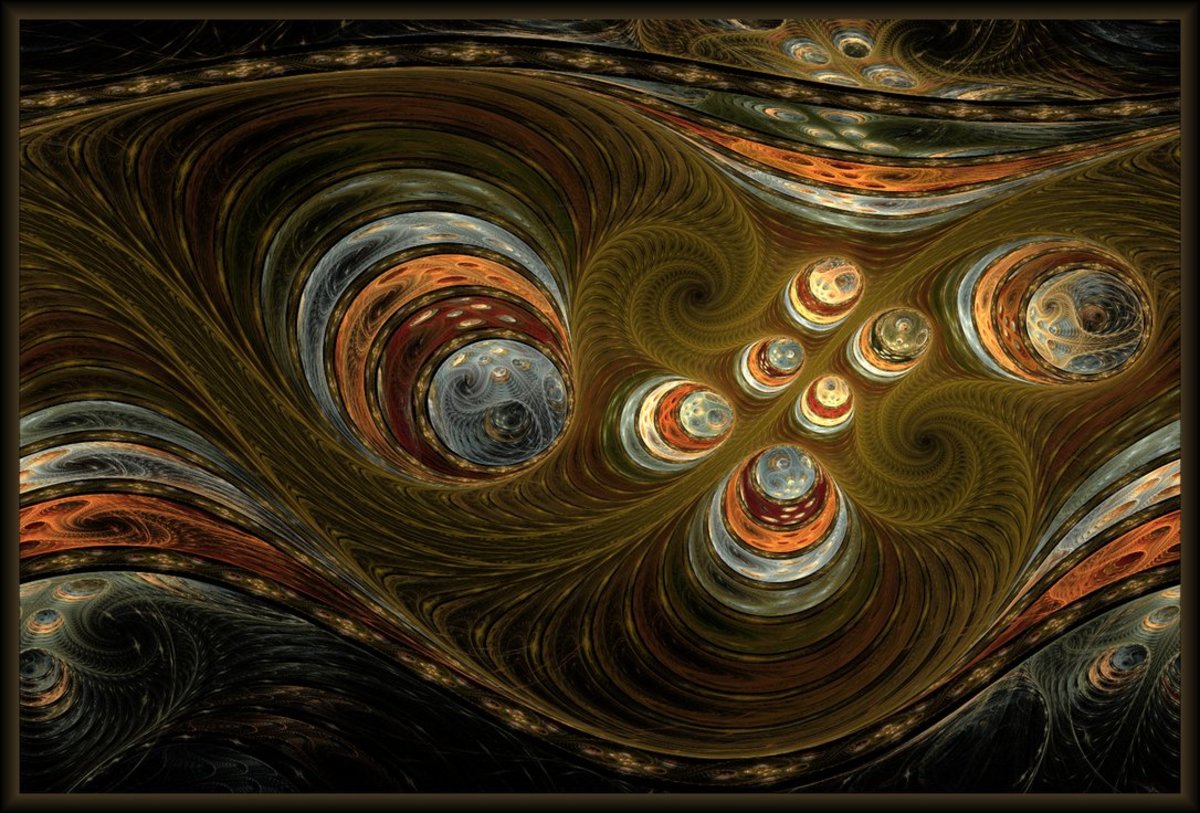This abstract digital illustration, possibly an oil painting, features a captivating cosmic scene set against a black backdrop, framed with a light white border. Dominating the left side of the image is a large, 3D stack of circular objects, culminating in a light blue orb. This stacks’ curved shape adds a sense of depth and movement to the artwork. To the right, a shorter yet similarly structured stack with an illuminated top orb mirrors the left stack, creating a balanced composition.

Flowing between these vertical structures are cascading swirls of gold, brown, and rust-red patterns, invoking the feel of swirling galaxies or black holes. These patterns, interspersed with smaller planets that seem to orbit on delicate, curved rings, contribute to the artwork's dynamic and ethereal nature. The rich interplay of colors, including blues, yellows, and deeper shades, spirals downwards and across the canvas, enhancing the sense of otherworldly motion and infinite space.